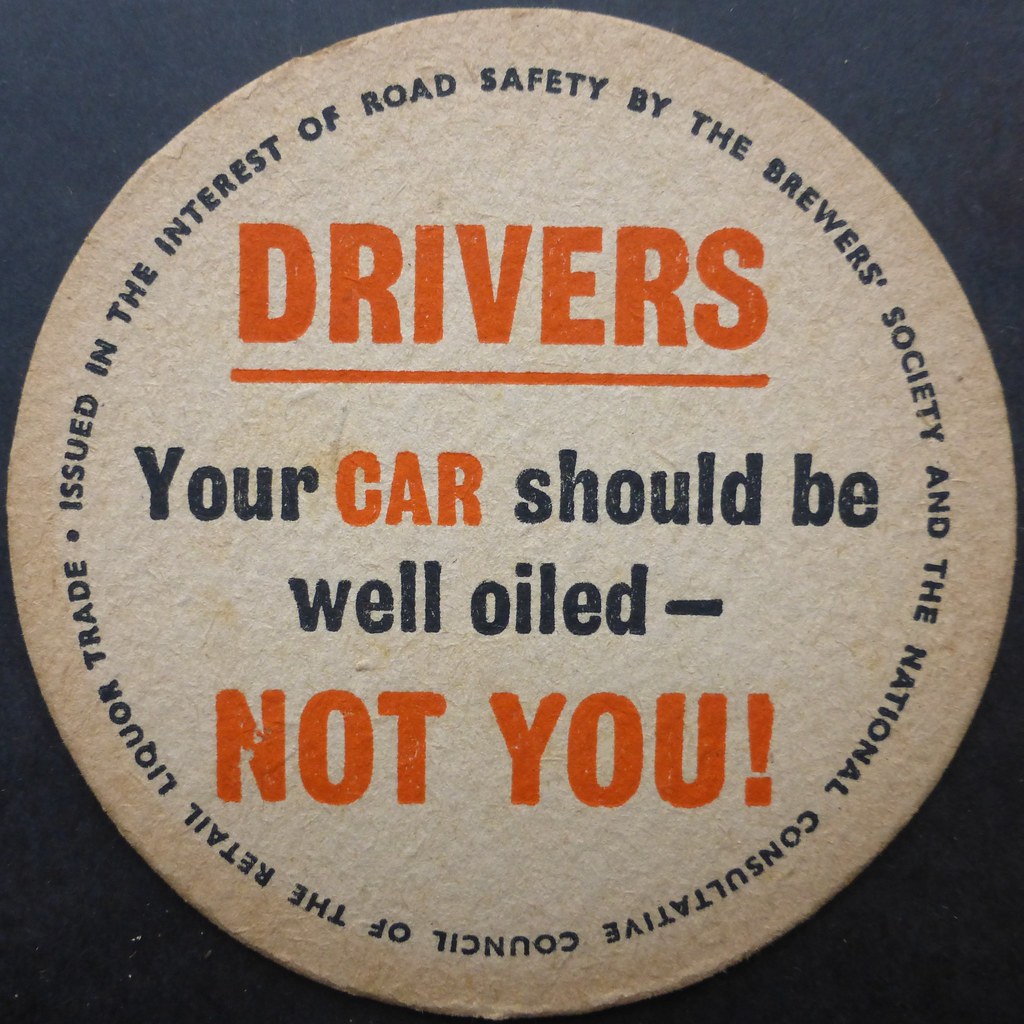The image features a close-up of an advertisement printed on a round, textured object resembling a coaster or fabric tag. The background is dark blue, almost navy, and matte. In the center of the circular object, set against a white backdrop, bold orange text reads "Drivers," which is underlined in orange. Below this, in black and orange text, it states, "Your CAR should be well oiled." Further down, in large orange letters, it emphatically declares, "NOT YOU!" with an exclamation point. Encircling the edge of the coaster in a circular fashion, black text reads, "Issued in the interest of road safety by the Brewer's Society and the National Consultative Council of the Retail Liquor Trade." The overall presentation suggests that it is an older or slightly faded promotional item advocating against drunk driving.